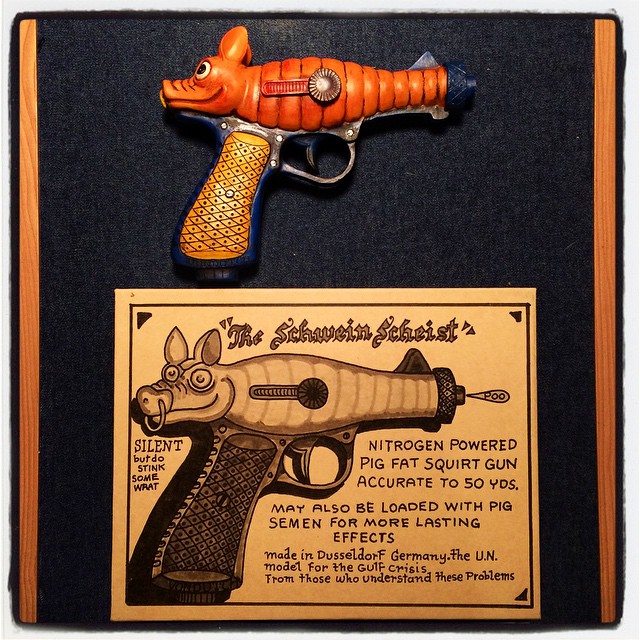The image depicts a close-up view of a museum display featuring a whimsical toy pistol named "The Schweinscheist." The gun, designed with a quirky orange pig as its barrel, rests against a black felt background bordered by two strips of brown wood. The handle of the gun showcases a yellow and black crisscross pattern adorned with small dots. The tip of the gun is textured in black. Below the pistol, a plaque provides a detailed description, reading: "The Schweinscheist. Silent but do stink somewhat. Nitrogen-powered pig-fat squirt gun, accurate to 50 yards. May also be loaded with pig semen for more lasting effects. Made in Dusseldorf, Germany. The UN model for the Gulf crisis, from those who understand these problems." The plaque features an illustration of the gun emitting a stream, potentially intended to resemble pig fat or an alternative substance.